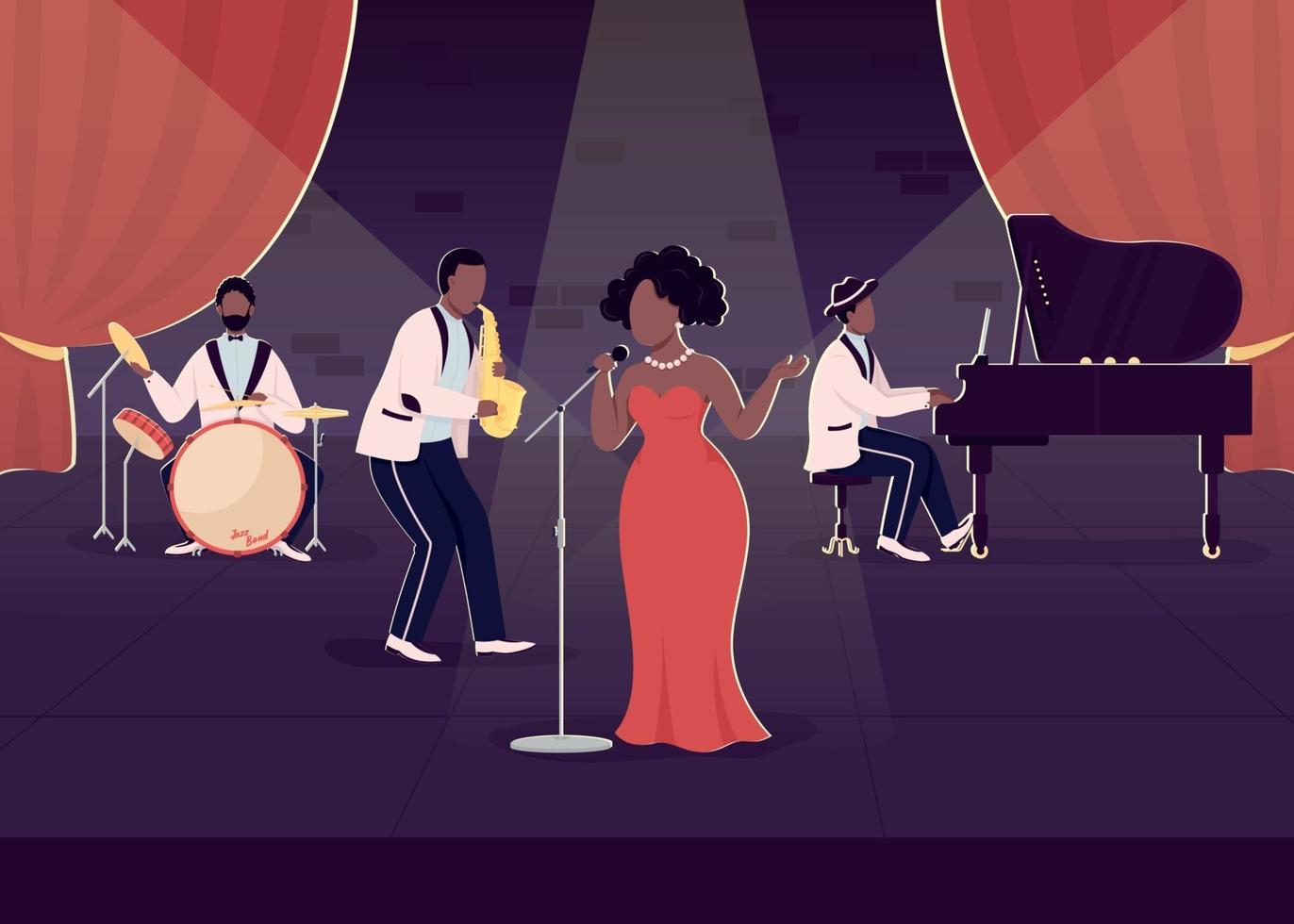The image is a vibrant, computer-animated, cartoon-like illustration of a jazz performance on a stage. The central figure is a black woman with short, thick, wavy hair, wearing a strapless, orange-red, full-length dress. She stands confidently at a microphone stand, her left hand bent at the elbow and extended upward, while her right hand grips the microphone. She accents her look with a white pearl necklace.

Surrounding her is an ensemble of three musicians. To her right sits a man at a black grand piano, attired in a white suit jacket over a light blue shirt, with blue pants, a black hat, and white shoes. On her immediate left is a saxophonist, similarly dressed in a white suit jacket, light blue shirt, black pants with a white stripe, and white shoes. At the far left of the stage is the drummer, who is also outfitted in the matching white jacket and black pants with a white stripe, accompanied by a light blue shirt and white shoes, and he is sitting in front of a tan drum set with orange trim.

The stage itself is adorned with large red curtains tied back with yellow ties, framing the background. The floor of the stage is purple, and illumination is provided by spotlights—two streaming in from the sides and one spotlighting the singer from above. The scene captures the essence of a classic, animated jazz performance with an emphasis on stylized, flat-shaded colors and features. None of the characters are rendered with facial features, contributing to the stylized and simplified aesthetic of the illustration.